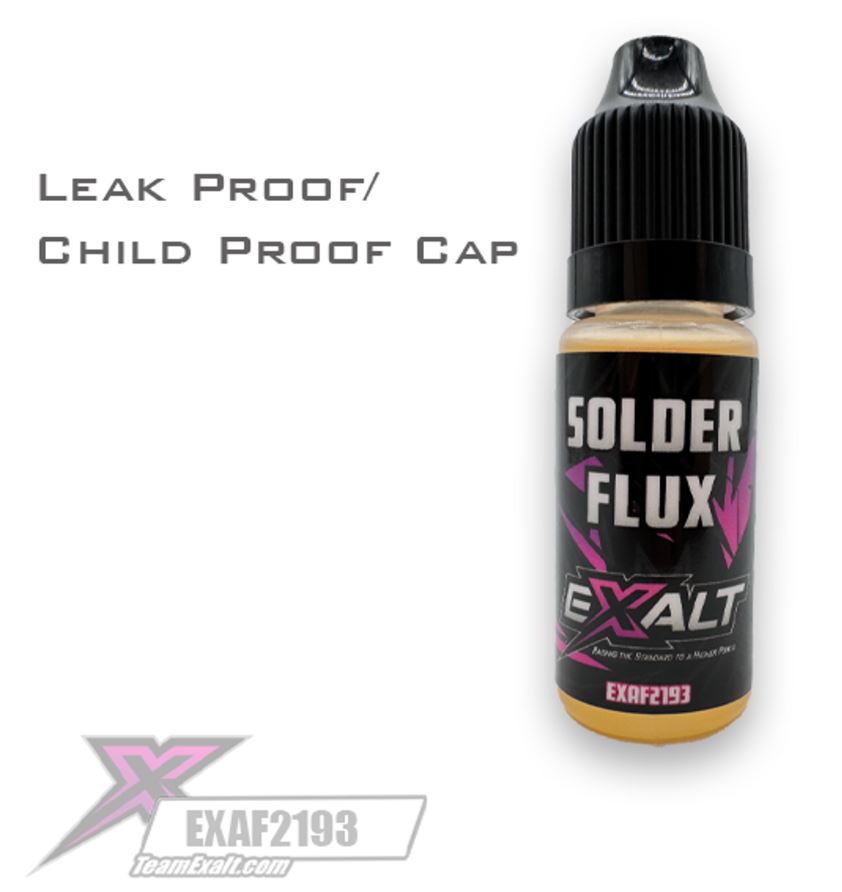This image showcases a product on a white background, prominently positioned on the right side. The product is a clear bottle with ridged, black cap containing a light beige liquid. The bottle's label is a combination of black and purple, with "Solder Flux" written in white font. Below this, the brand name "Exalt" is also in white, but its "X" is distinctively pink or purple. At the very bottom of the label, the product code "EXAF2193" is displayed. 

On the left side of the image, the top text reads "leak-proof/child-proof cap" in gray letters. In the lower-left corner, there is a standout pink "X," followed by the product code "EXAF2193," and the URL "teamexalt.com" in a banner format. The cohesive focus on labeling highlights the product's child-proof and leak-proof features, emphasizing both functionality and brand identity.